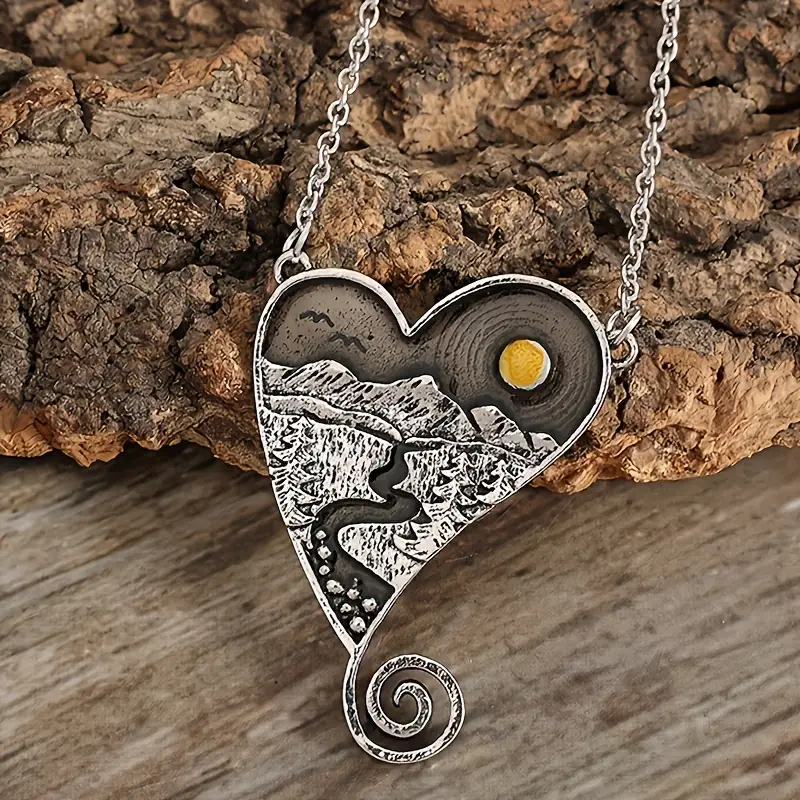This image features a meticulously crafted, heart-shaped pendant necklace placed delicately on a wooden, rocky surface. The pendant itself is made of metallic silver and showcases an intricate landscape encapsulated within the heart. On the left upper quadrant of the pendant, two birds are gracefully flying, and on the right upper quadrant, a golden sun or moon glows. Below this, detailed engravings of mountains and a river, or pathway, winding down to the base of the heart are depicted. Adding to its charm, the bottom of the heart extends into a swirling, spiraled design. The silver chain, visible on both sides of the necklace, complements the overall delicate aesthetic of this exquisite jewelry piece. The light brown and dark brown hues of the background rocks contrast beautifully with the pendant's silver and black tones, highlighting its intricate details and craftsmanship.